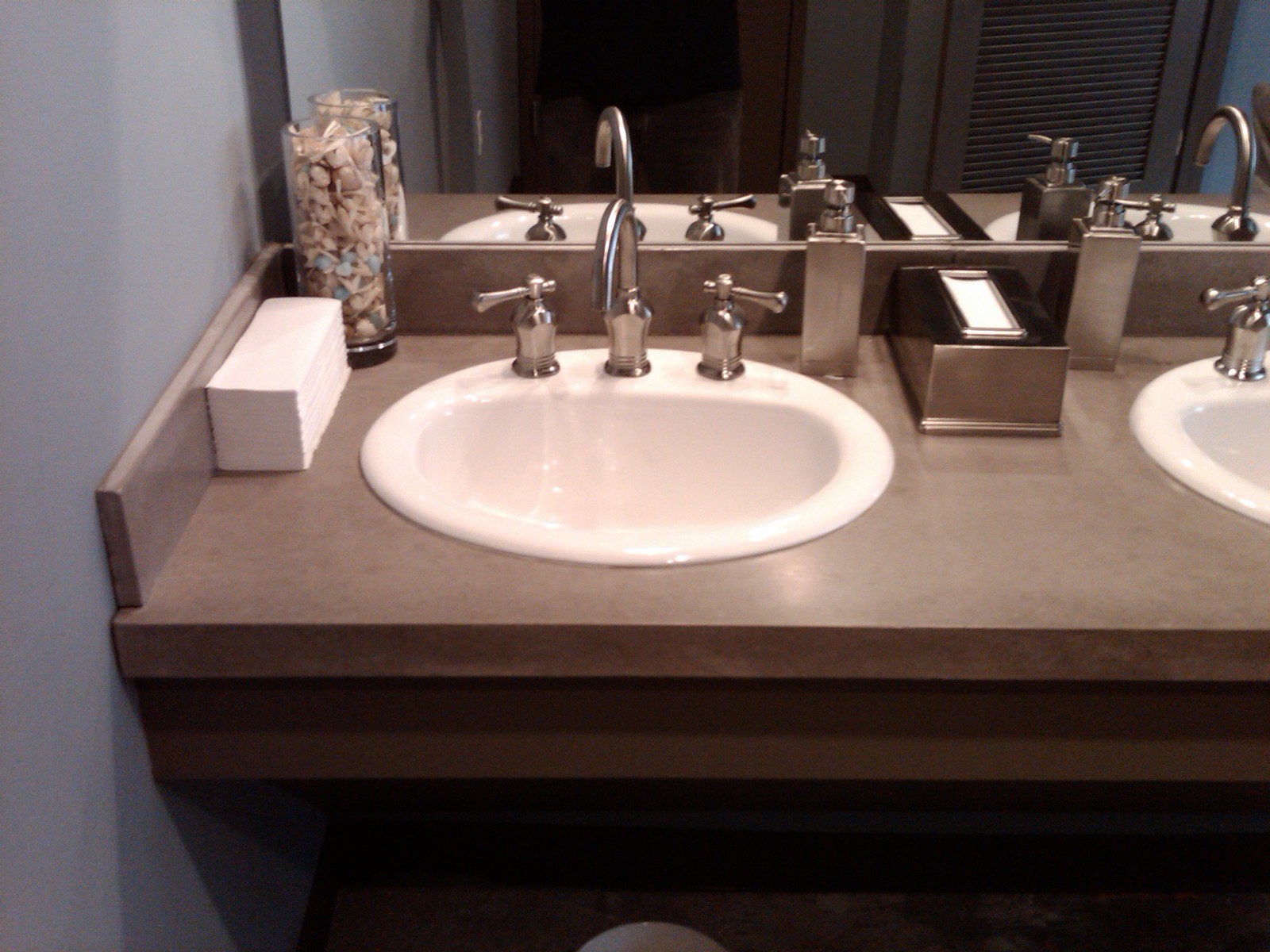This photograph captures a meticulously arranged restroom scene, which could be either in a residential or commercial setting. The focal point is a vanity top featuring two sinks with gleaming chrome faucets. Between the sinks, a chrome-plated tissue holder is prominently displayed. Adjacent to each sink, there are stainless steel or chrome-coated soap dispensers, ensuring convenience and hygiene. To the far left of the image, a stack of C-fold paper towels is neatly placed for drying hands. Adding a touch of elegance, a decorative glass decanter sits to the side, filled with white objects that appear to be potpourri or possibly seashells, enhancing the aesthetic appeal of the space. The overall ambiance of the restroom exudes cleanliness and sophistication.